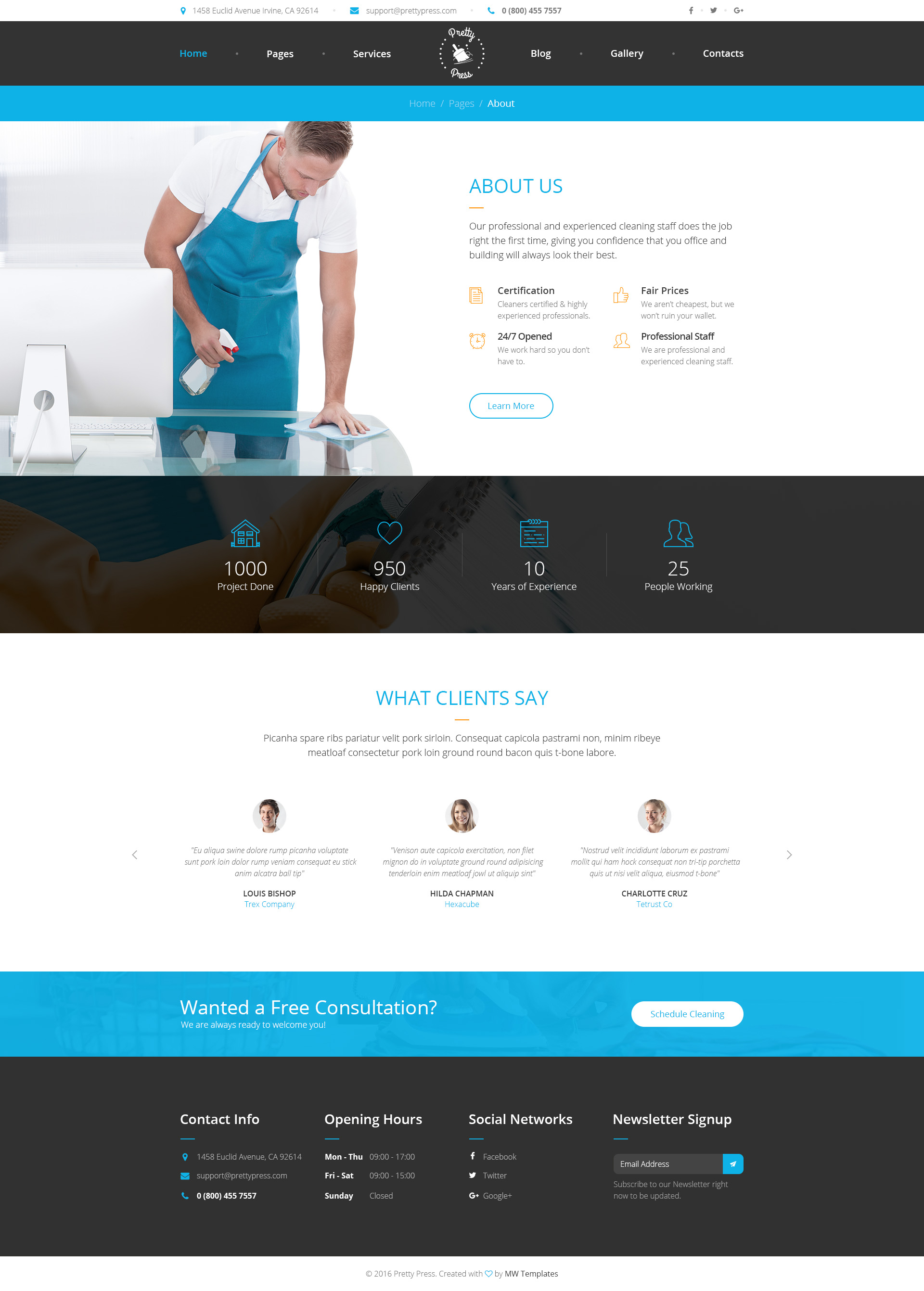The image depicts a webpage with a black header at the top featuring the words "Services," "Gallery," and "Contact." Beneath this header, there is a blue border. The main image displays a person wearing a short-sleeved shirt and a blue apron, holding a spray bottle and a rag, wiping a table. This section is titled "About Us," followed by an indistinct block of text that is too blurry to read clearly. Below, numbers such as "1,950," "10," and "25" are visible, under a section titled "What Clients Say," accompanied by a couple of paragraphs. Further down, there is a blue box prompting users to "Request a Free Consultation." The bottom of the page features a black box containing sections labeled "Contact Info," "Opening Hours," "Social Network," and "Newsletter Signup." The rest of the content is too small and blurry to discern.